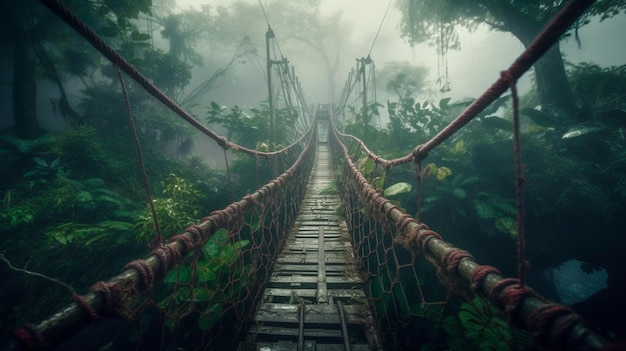The image illustrates the entrance to a rope bridge set within a dense, mystical rainforest. Enveloped in fog and mist, the scene exudes a haunting, fairy-tale-like ambiance. The bridge itself is made of wooden planks, some of which are missing, exposing precarious gaps that enhance its fragile and rickety appearance. The sides of the bridge are secured with ropes, and there's a distinctive red netting visible along the edges. Lush greenery surrounds the bridge, with a variety of large leaves and different plants, including towering trees and lower vegetation. The perspective suggests the viewer is standing at the start of the bridge, looking into the misty depths of the jungle, which further adds to the eerie and enchanting atmosphere. The overall effect is ethereal, with a smoky, cloudy feel and a vignette effect framing the illustration, enhancing its dreamlike quality.